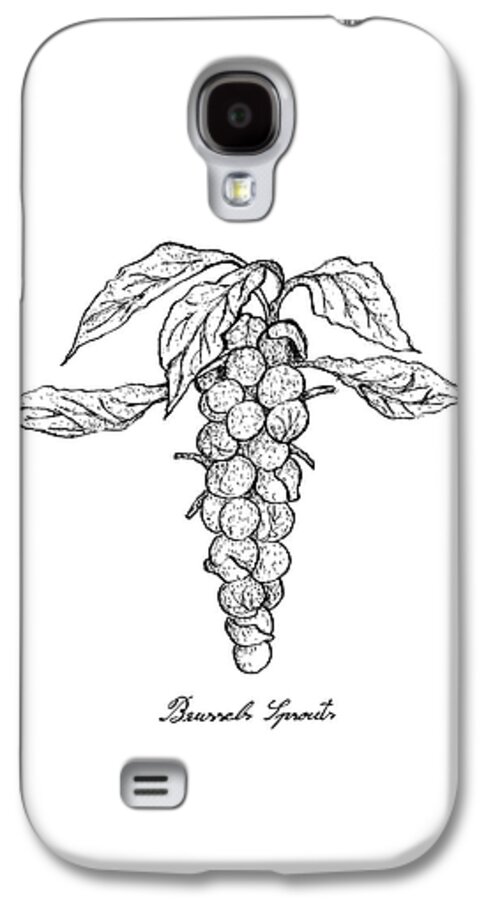The image depicts a white cell phone case adorned with a detailed black and white illustration of Brussels sprouts. Positioned near the top, the case features a cutout for the camera. The Brussels sprouts illustration starts with large leaves at the top and cascades down in a bunch, resembling the shape of a grape cluster, with individual sprouts tapering off towards the bottom. Beneath this artistic rendering, the words "Brussels Sprouts" are elegantly inscribed in a cursive script that evokes a historical feel, similar to the handwriting of Thomas Jefferson. Additionally, there is a small rectangular cutout in the lower left corner, presumably for the phone's speaker. The case, resting against a white background, has a slight ivory glow, adding a sophisticated touch.